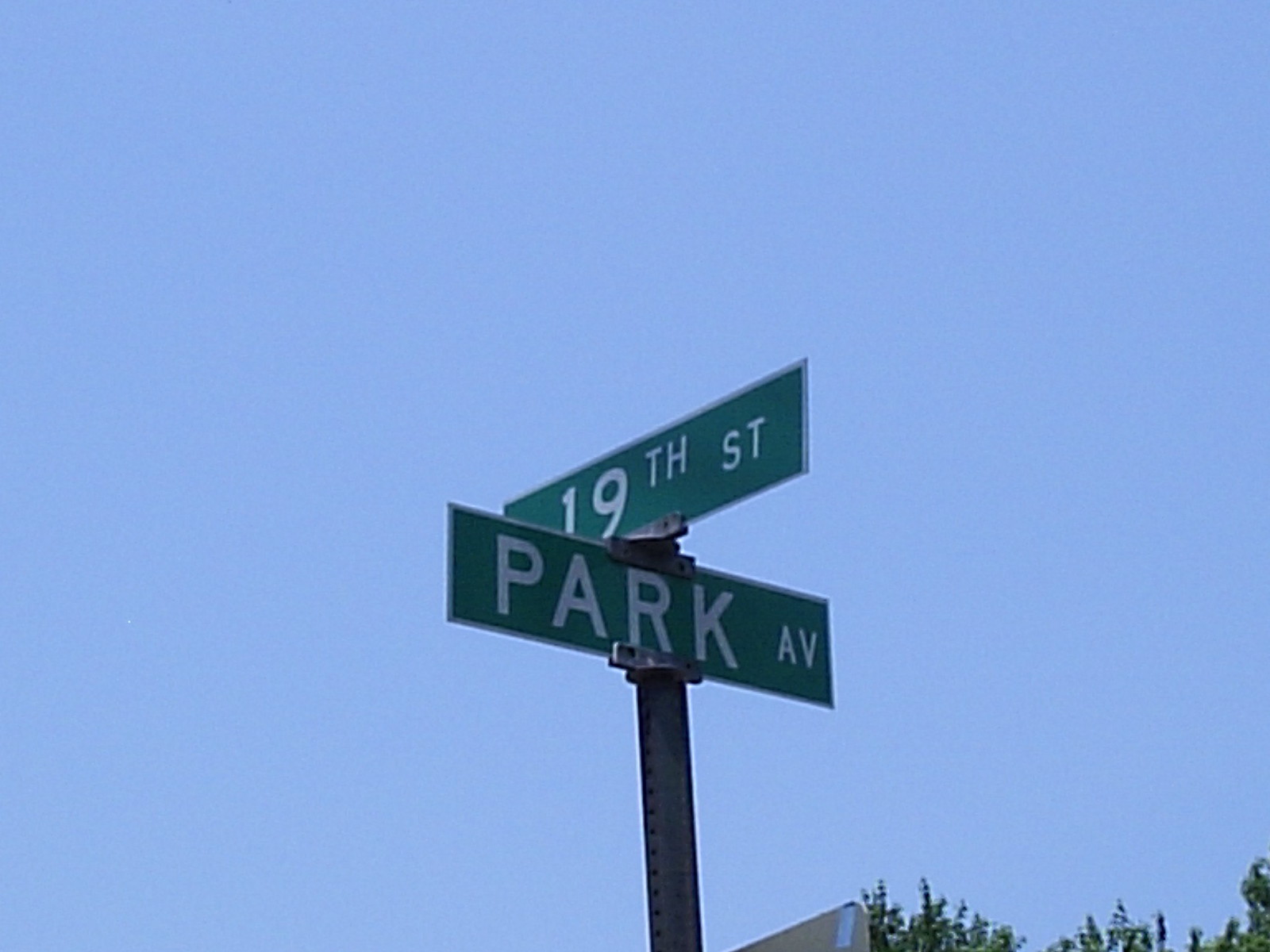In this image, we see a street sign at the intersection of Park Ave and 19th Street, set against a clear light blue sky. The shot is taken from below, looking upwards, with only the tips of trees peeking into the frame. On the right side, there are a few green leaves from side-by-side trees. To the left, there's a slight appearance of brown foliage. The street sign is mounted on a gray post and features two green rectangular signs with white text. The lower sign reads "Park Ave," while the upper sign reads "19th St." The serene background highlights the minimalistic details of the street intersection.